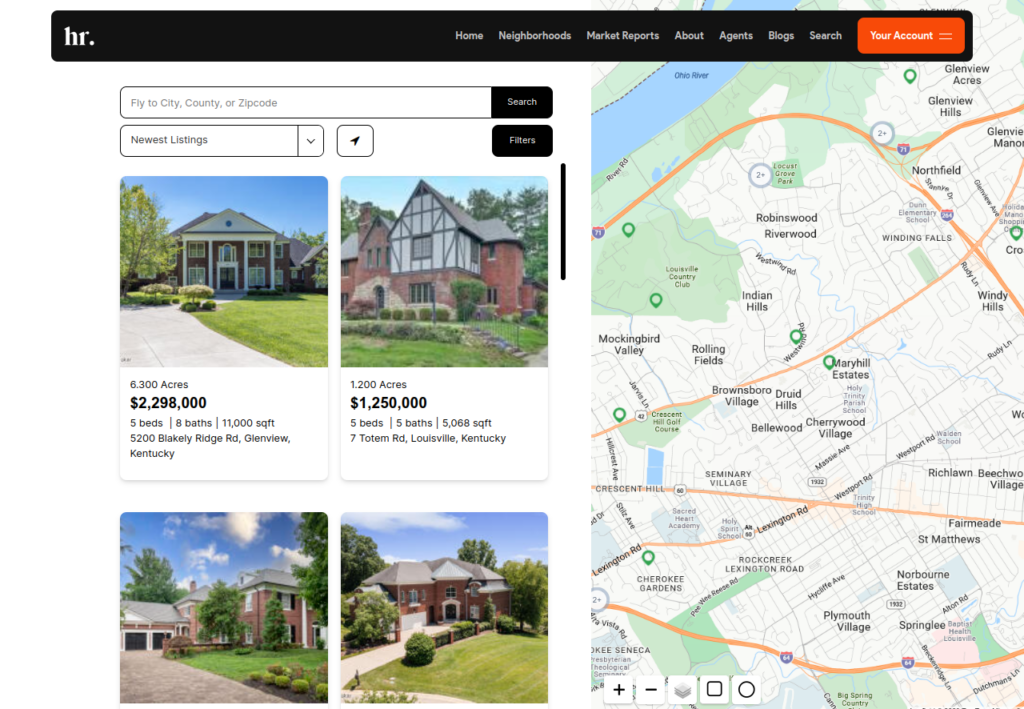The image is a rectangular web interface with its longer side extending horizontally. It features a black header with white text, where "HR" appears on the top left corner. Towards the center to the right, the header lists menu options: Home, Neighborhoods, Market Reports, About, Agents, Blogs, and Search. An orange, reddish-orange button labeled "Your Account" with white text is positioned adjacent to these menu options.

Below the header, the layout divides into two sections. The left section allows users to search for properties by city, county, or zip code, with "Newest Listings" pre-selected. Underneath this search panel, images of four homes are displayed. The top two homes are distinctly showcased with detailed information. The first home, located on the left, is in Louisville, Kentucky, featuring 6.3 acres, five bedrooms, six bathrooms, and an 11,000 square foot area. The second home, on the right, covers 1.2 acres with five bedrooms, five bathrooms, and a 5,000 square foot area.

The right section of the image presents a map, presumably highlighting the searched area, although the specific city isn't explicitly clear. This map aids users in visualizing the locations of prospective homes, emphasizing the purpose of the interface in helping users find properties for rent or purchase.